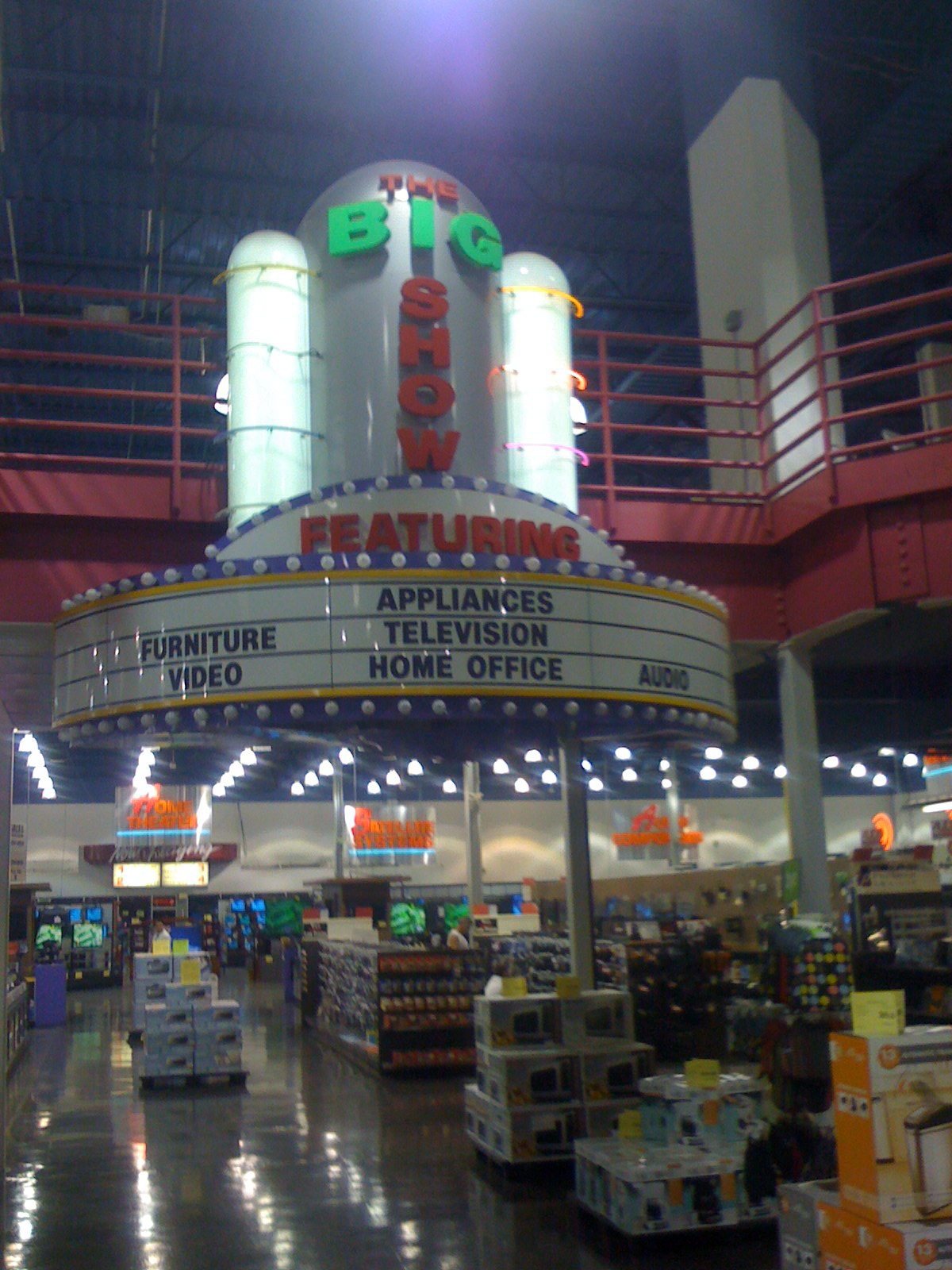The photograph captures a display inside a spacious, semi-industrial store with an open warehouse aesthetic. The store features an upper loft-type space that serves as a centerpiece for a striking display with a cinematic theme. Mimicking the facade of a vintage movie theater, the display boasts a light-up marquee adorned with various product categories including "Furniture," "Video," "Appliances," "Television," "Home Office," and "Audio." Above the marquee, lighted cylindrical sections add to the theatrical ambiance. At the center, in bold letters, "The Big Show" is prominently displayed, encapsulated by an array of round lights that, though currently unlit, promise a visually captivating experience when illuminated. The overall effect is a nostalgic nod to classic theater design, seamlessly blending commerce with a touch of Hollywood glamour.